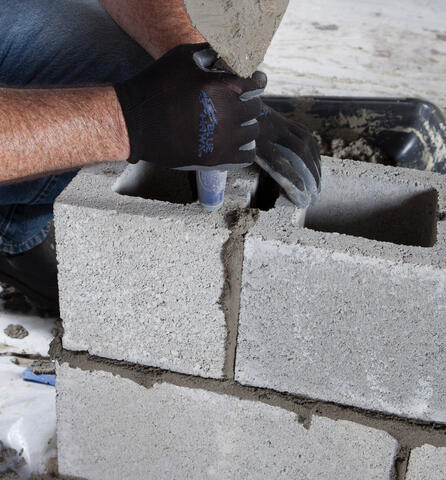A man, dressed in jeans and a grayish t-shirt, is deeply engaged in masonry work, constructing a wall with cinder blocks on what appears to be a stone floor partially covered by a plastic tarp. His exposed, hairy forearms hint at his physical effort as he crouches down, wearing black and gray work gloves. Using a grayish-blue tool in his right hand, which seems to dispense a dark gray cement or mortar paste, he carefully aligns and secures a half cinder block to a full one, ensuring a firm bond. His left hand stabilizes the blocks, pressing them together to form the edge of the wall. In the background, the scene is subtly defined by a blurred gray ambiance and a partially visible black plastic bucket, adding context to his meticulous labor.